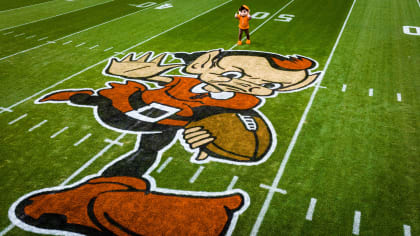This image showcases the central section of a football field around the 50-yard line. Dominating the scene is a detailed painting of a leprechaun-like football player positioned prominently in the middle of the field. The leprechaun character is depicted with pointed ears, a pugnacious face, and a short crop of orange hair. Dressed in an orange tunic reminiscent of 17th-century attire, it also sports a belt with a white buckle, brown pants, and distinctive orange shoes. The leprechaun is holding a large football in one hand and has its right arm extended in a stiff-arm pose typical of a football player. Complementing this painted character, the actual team mascot stands just above the artwork, dressed identically with an orange hat, shirt, belt with a white buckle, black pants, and orange shoes. The photograph captures the mascot from an aerial perspective, making the actual person appear small in comparison to the painted figure. The well-maintained green grass and white yard lines of the football field provide a vivid background to this scene, emphasizing both the painting and the live mascot.